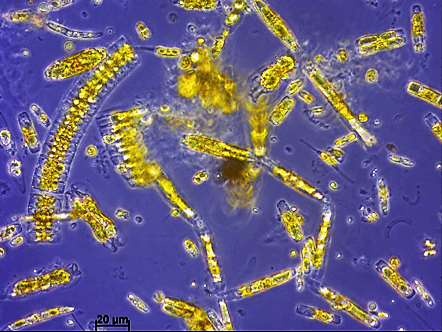This detailed image depicts a dark blue, almost purple, background filled with various bizarrely shaped yellow forms that resemble bacterial cells under a microscope. Among these are an assortment of circles, triangles, squares, oblong shapes, and even some ambiguous forms that look like snakes or railroad tracks. These yellow shapes, distributed randomly across the image, include both small and large rods, double circles, ovals, and other irregular configurations. The center of the image is marked by a conspicuous black splotch and a blurry, shapeless yellow mass above it. Scattered throughout the background are small white capsules, as well as semicircular patterns adding to the complex visual array.